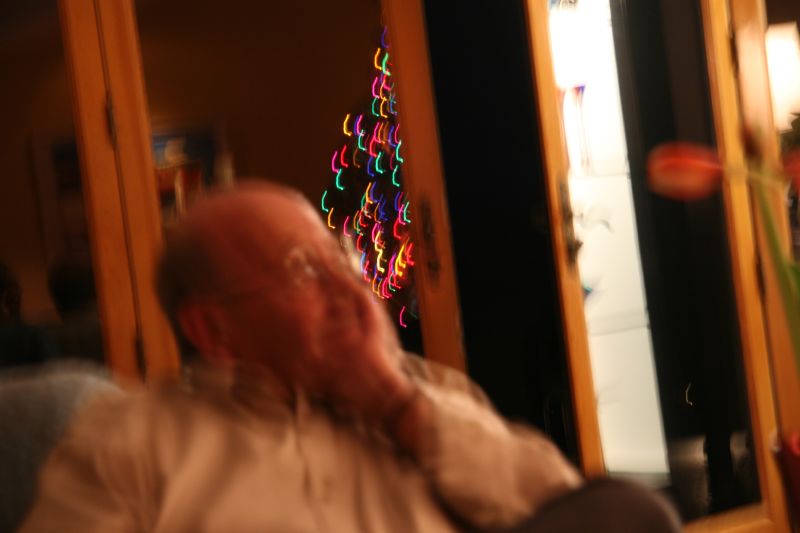This is a very blurry photograph capturing an elderly man, presumably a grandfather, enjoying Christmastime. Positioned in the left middle foreground, he is seated on a chair or couch. The man, who appears to be balding with dark gray hair, is wearing glasses and a white collared shirt paired with gray or possibly brown pants. He has his hand thoughtfully resting on his chin. The festive season is indicated by a Christmas tree situated in a different room behind him, discernible by the colorful array of blue, light blue, green, red, orange, and yellow Christmas lights. Also in the background is a door with a glass pane and a tall, floor-standing mirror to its right, adding depth to the scene. Despite the blurriness, the image evokes a sense of holiday warmth and familial comfort.